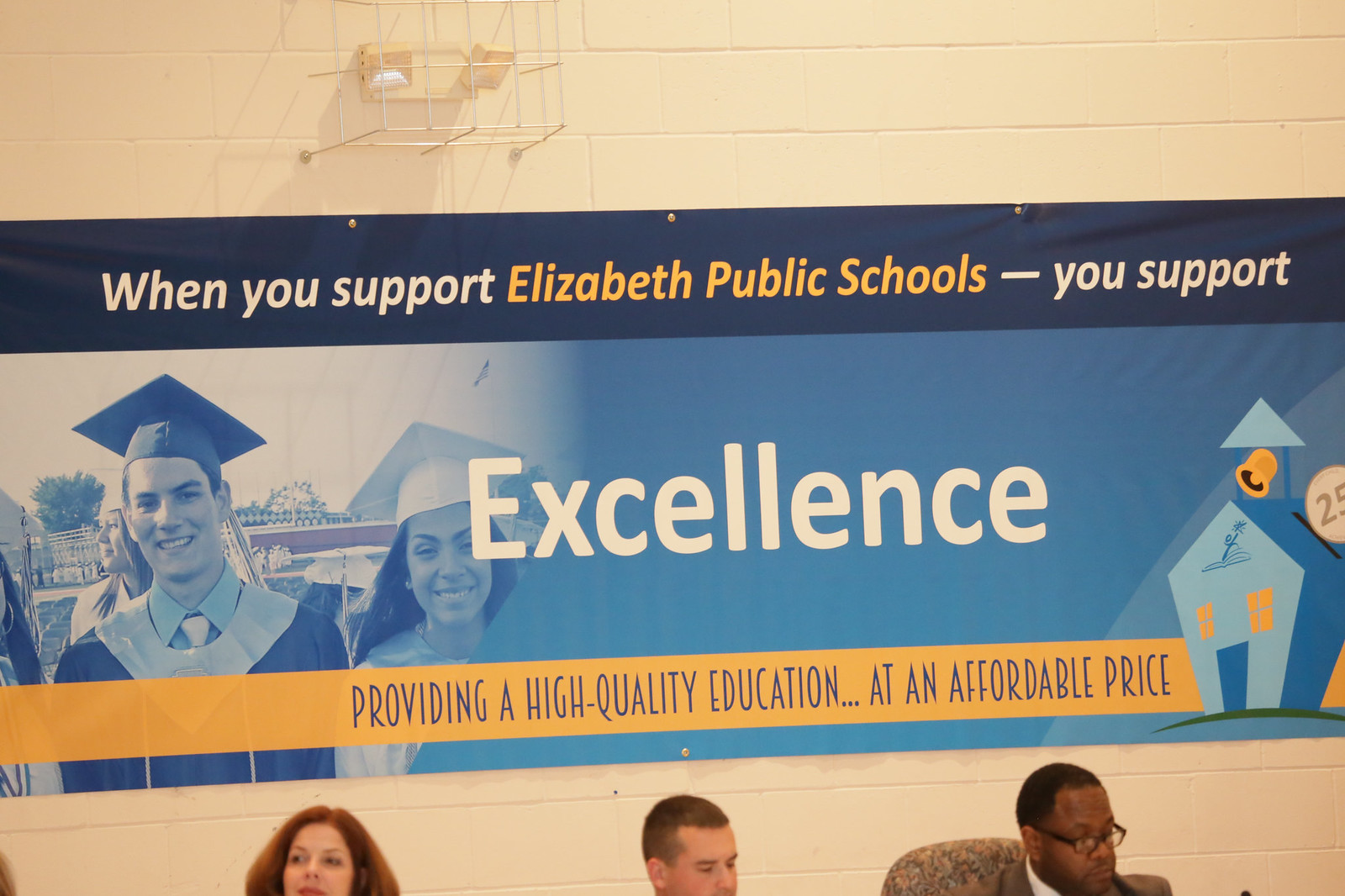This detailed horizontal rectangular photograph captures a moment during a school board meeting, held in what appears to be a room adorned with a wall mural and a prominently displayed poster. The poster, primarily blue in color, features a darker blue band at its top with white and yellow lettering that reads, "When you support Elizabeth Public Schools - you support." This leads into the middle portion of the banner where, in large white letters against a blue background, the word "excellence" is boldly displayed. To the left of "excellence," there are images of two students in graduation attire, one male and one female, symbolizing academic achievement. On the right, there is a cartoon character and what seems to be an odd-shaped school door.

Below this, a yellow band with blue and yellow print states, "Providing high-quality education at an affordable price." In front of the mural and poster, three individuals are seated at a table. On the left is a woman with red hair, looking to her right. In the center is a man with a crew cut, glancing to his left, and on the right, a black gentleman with glasses, sitting on a cloth-backed chair, is looking down. This image vividly captures the elements of the school board meeting and the educational values promoted by the Elizabeth Public Schools.